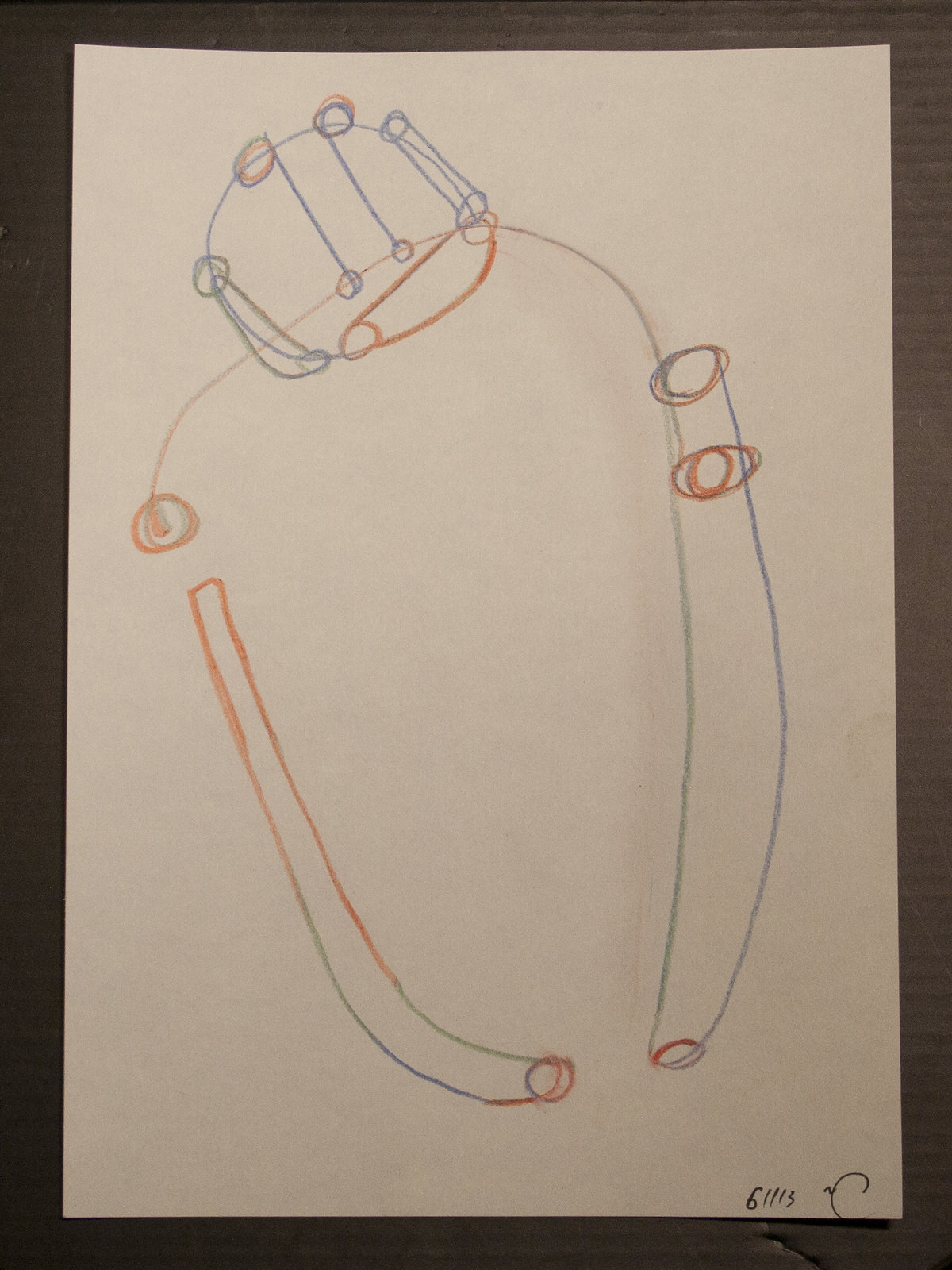A children's drawing is depicted in the image, created on an approximate 8.5 by 11-inch sheet of slightly off-white manila paper, leaning towards a craft brown hue. This paper rests atop a dark brown table, evidenced by the slightly lifted corners. The focus of the drawing appears to be a simplistic representation of a robot. The robot's head is portrayed as a large circle with additional smaller circles adorning its edge, accompanied by an oblong-shaped mouth within it. Below the head, a single line arcs downward, resembling shoulders. Extending from these are two disproportionately long, unattached arms; the arm on the drawing's right side connects at its base to the curved shoulder line. Both arms feature circular elements at their extremities. The drawing employs a minimalistic color palette of orange, blue, and green. In the bottom right corner, there is an inscription or name, though it is mostly illegible.